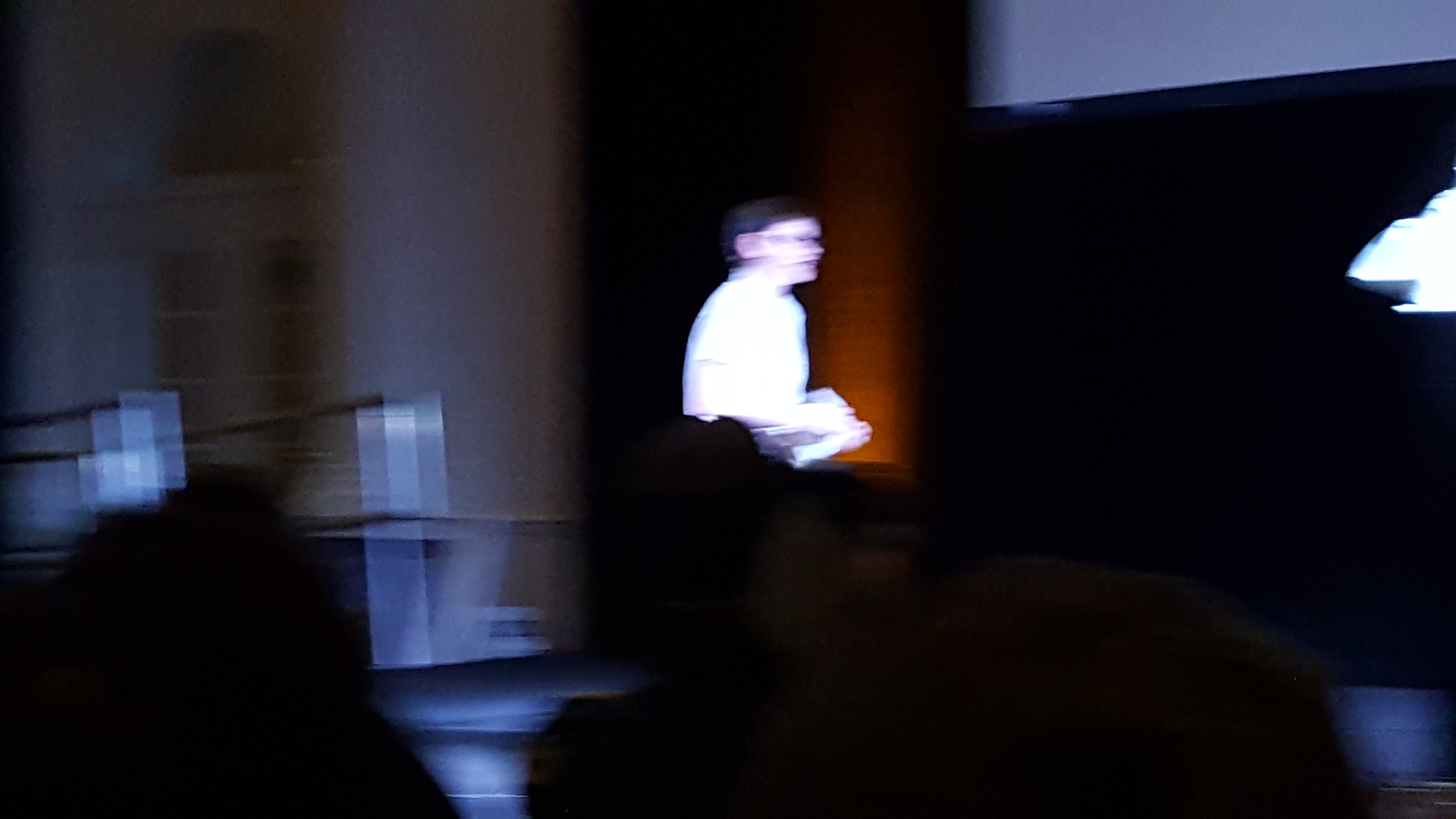This horizontal image is challenging to interpret due to its blurriness. It seems to capture a moment from a school event, likely held in a dimly lit auditorium. In the lower foreground, the silhouettes of adults' heads are faintly visible, suggesting the photo was taken from within the audience. Central to the image is a young boy with short brown hair and glasses, dressed in a light-colored shirt. He is holding a book and facing to the right. The event could be a school play or another type of performance. The background on the left side is dark brown and appears to include rectangular glass or plastic containers. The right side of the photo fades into a large black area, contributing to the overall obscurity of the scene.